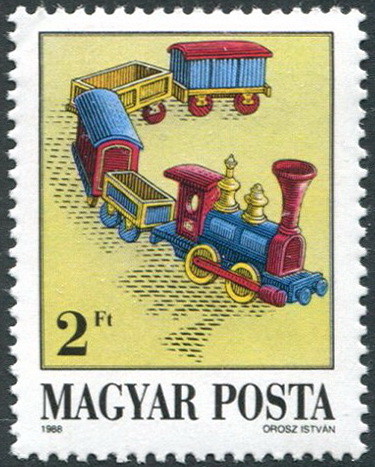This is an image of a 1968 postage stamp with a white perforated border, set against a black background. The central image is an artistic drawing of a colorful old train, possibly a toy train, featuring a blue engine with red and gold accents. The engine, specifically, has a red cab, a red steam pipe, and two gold whistles. The wheels are outlined in yellow, with a red drive bar. The train also includes a blue coal car outlined in yellow, a red boxcar with a blue roof, another yellow open box trailer with red wheels, and a final red-wheeled, yellow-bottomed blue boxcar with a red roof. On the stamp, there is a yellow square containing the train image, and beneath it are the words "Magyar Posta" and "Oroz Istvan" in black text, indicating its Hungarian origins. The denomination "2FT" and the year "1968" are also visible, emphasizing its collectible nature.